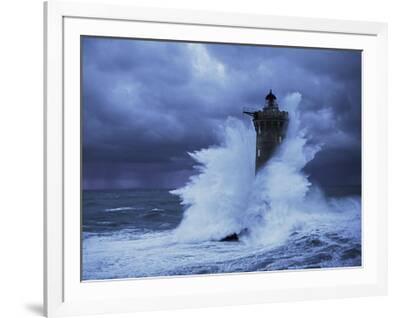The image is a framed print of a photograph displayed at an angle, presenting a stormy seascape. The photograph, enclosed in a layered white frame, showcases a small yet dramatic scene of a dark, tumultuous ocean under a gray, cloud-heavy sky, evoking a sense of a dreary, stormy day. Central to the image is a cylindrical, dark gray lighthouse, characterized by its tower shape with a narrow top and several windows, standing resolutely amidst the crashing waves, which surge nearly to the top of the structure. The lighthouse's light is either faintly illuminated or not visible due to the storm conditions. The scene vividly captures the ferocity of the sea, with towering waves and thick clouds dominating the composition.